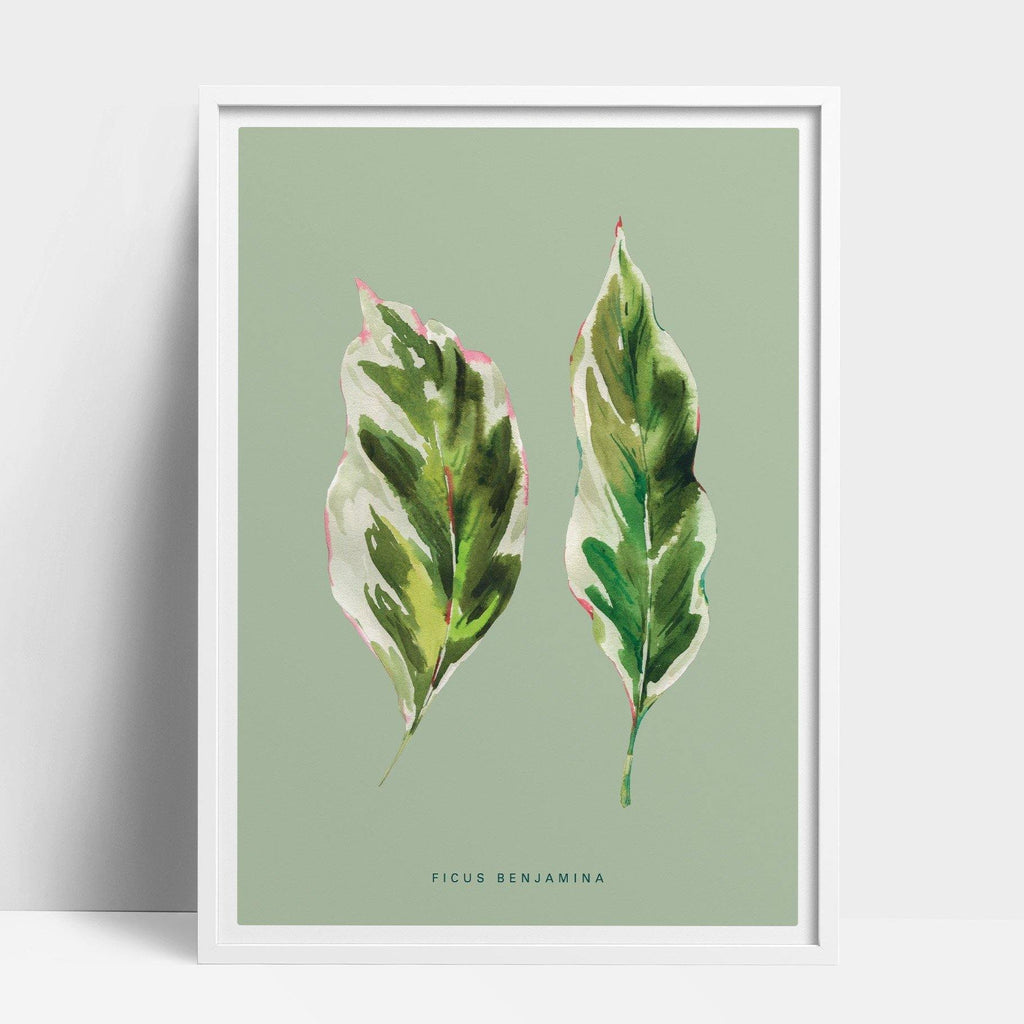The artwork in question is a delicately crafted watercolor painting of two Ficus Benjamina leaves, framed within a plain white border. The leaves are set against a soft, sage green background that complements their natural hues. The leaf on the left is short and broader, featuring a gradient from dark green to white with pink tinges at the tips. The leaf on the right is thinner and slightly longer, similarly transitioning from green to white with hints of pink at the top and bottom left. Both leaves are detailed with elongated, thin, and delicate stems. At the bottom middle section of the artwork, the name "Ficus Benjamina" is inscribed in black text, providing a clear identification of the depicted plant species.